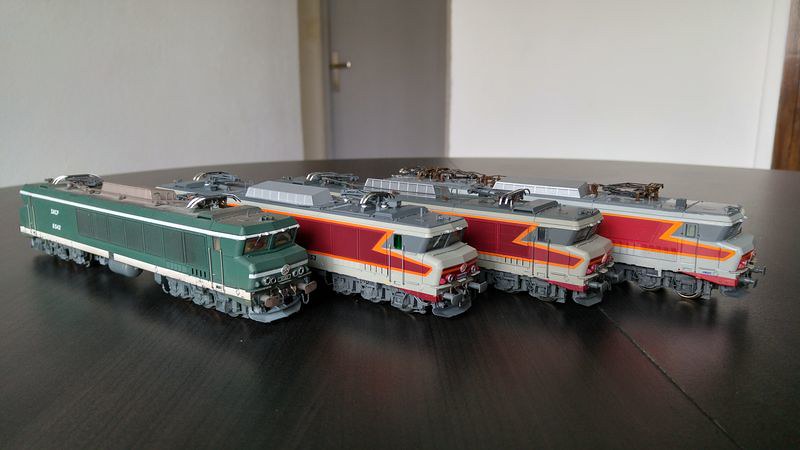In this image, we see a collection of four model train engines meticulously arranged on a dark brown, round wooden table. The room is minimally furnished, featuring stark white walls and a gray door with a metallic handle. The detailed description of each train engine highlights their distinct features: 

The first engine, positioned on the left, is predominantly dark green with white stripes at the top and bottom and beige access panels on the roof. It sits on gray wheels, typical of train tracks. The next three engines are identical, predominantly off-white with striking dark red zigzag patterns bordered by orange on their sides. Their roofs and various components are colored in shades of gray and silver. 

Additional details include the seamless appearance of the round table, which has a central line suggesting it might expand with a leaf, and the overall simplicity of the room that directs full attention to the detailed model trains.